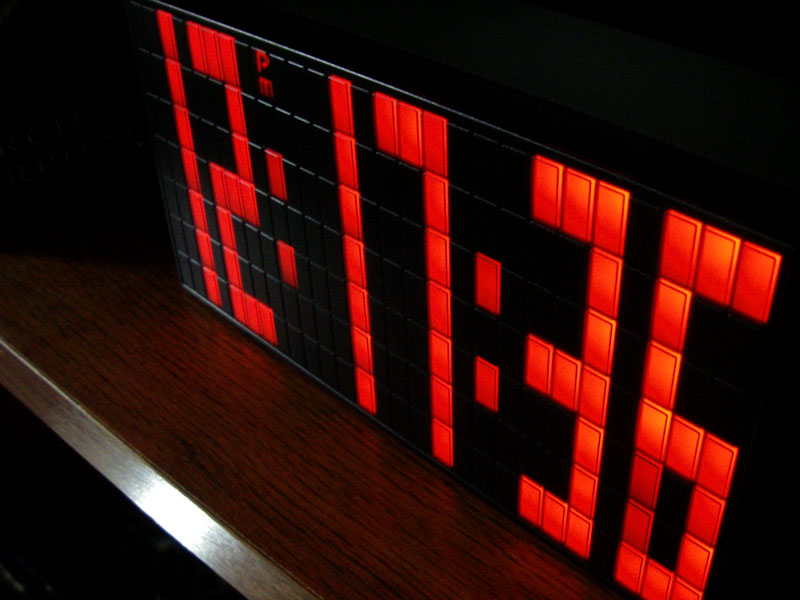This is a close-up photograph showcasing a digital clock, captured in a slightly rectangular, landscape format. The shot is taken from an angle, orienting the clock upwards and to the left, highlighting its sleek, black casing adorned with a pattern of small black squares. The time displayed on the clock reads 12:17:36 PM, illuminated in a vivid orangish-red hue. The clock rests on a dark brown wooden table, which is complemented by a silver frame.